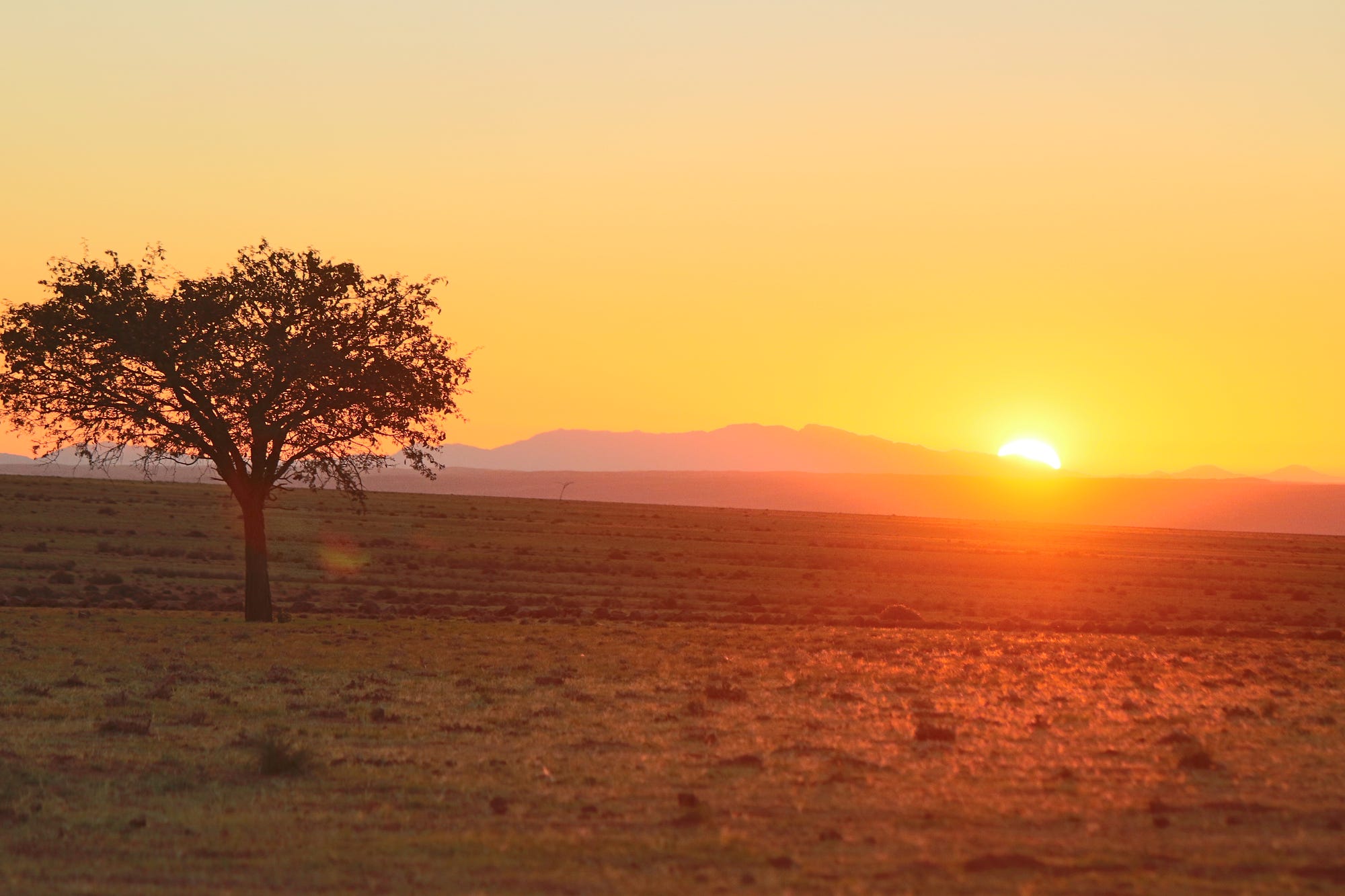This captivating photographic image captures the serene beauty of a desert landscape during sunset. The setting is an austere, open plain with a barren, sandy foreground that dominates the lower third of the image. In the background, centered and stretching across the horizon, is a series of hazy blue mountains. The sun, a bright yellow orb, is partially visible as it sets behind these mountains, contributing to a stunning palette of colors in the sky and landscape.

The sky is a gradient of warm hues; immediately around the sun, it radiates a vibrant yellow, transitioning into shades of orange, peach, and, finally, a soft gray at the top of the image. On the far left section of the photograph is the silhouette of a single tree, which stands out against the warm backdrop. This tree, with its high trunk splitting into three or four branches adorned with leaves, casts a striking black shadow. Scattered sparsely across the savanna-like plain are small shrubs, with possible distant trees blending into the landscape.

Despite the barrenness of the desert soil in the foreground, the vivid colors of the sunset and the lone tree silhouetted against the sky evoke a quiet, profound beauty. No text disrupts the visual storytelling, allowing the viewer to fully immerse themselves in the natural tranquility of this compelling outdoor scene.